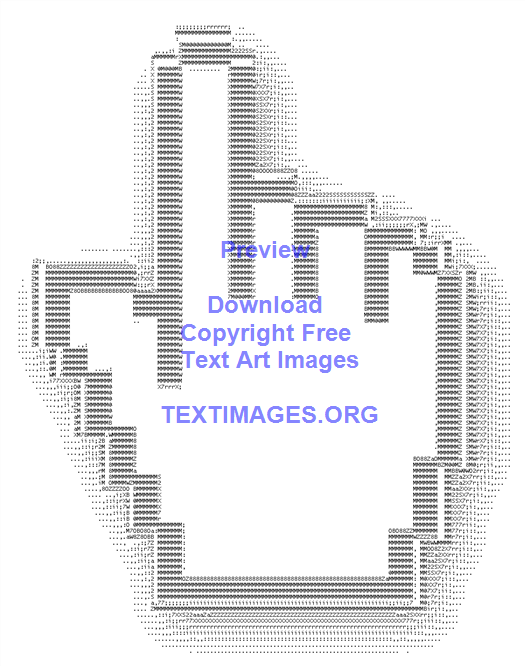The image depicts a digital representation of a right hand made entirely of numbers and symbols, giving it a pixelated appearance. The hand is pointing up with the index finger extended and the thumb outward, while the remaining fingers are bent down, reminiscent of a foam finger often seen at sports events. The hand itself is white and set against a background that transitions from black to gray, creating a shadow effect around the edges. Blue text appears within the hand, stating "preview, download copyright free text art images," followed by "textimages.org" in all caps. The intricate design uses numerous sequences that blend together, too fine to distinguish the individual symbols clearly from a distance.